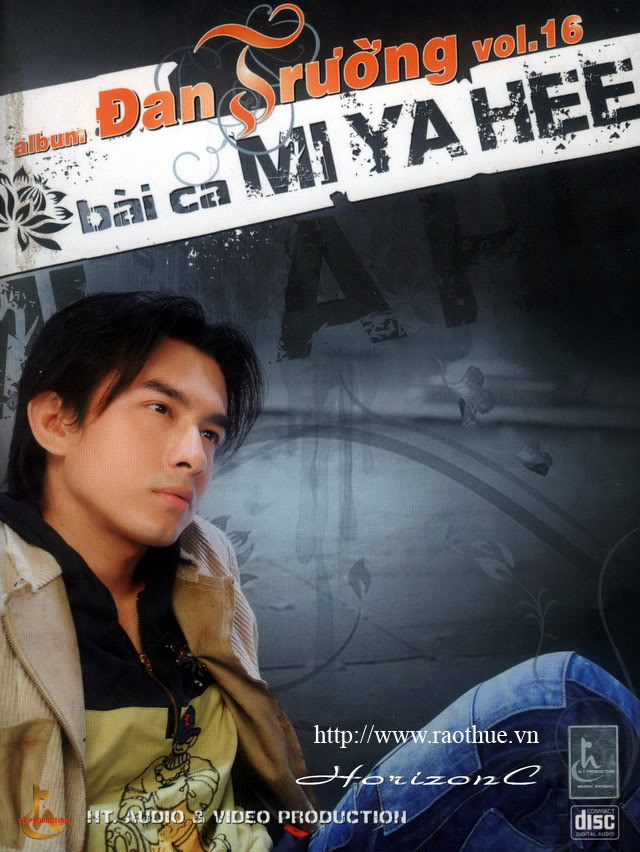The image is a detailed cover art likely for a music album. At the top of the cover, stylized text reads, "Album Dan Sreeyong Volume 16 by Ka Miyagi," showcasing a combination of lowercase and capital letters along with a small lotus design. Seated in the foreground is a young man of Asian descent, appearing to be around 22 years old. He exudes a contemplative, somewhat brooding demeanor as he gazes wistfully into the distance. The man is dressed in a mixed dark and light brown jacket layered over a t-shirt featuring a cartoonish design. His outfit is completed with jeans made of various patches. Against a grayish background, the entire scene is imbued with a subtle, melancholic vibe. Toward the bottom of the image, additional text, "www.raothue.vn," is written over the man's figure, providing a possible Vietnamese connection, and indicating the website might offer further information.